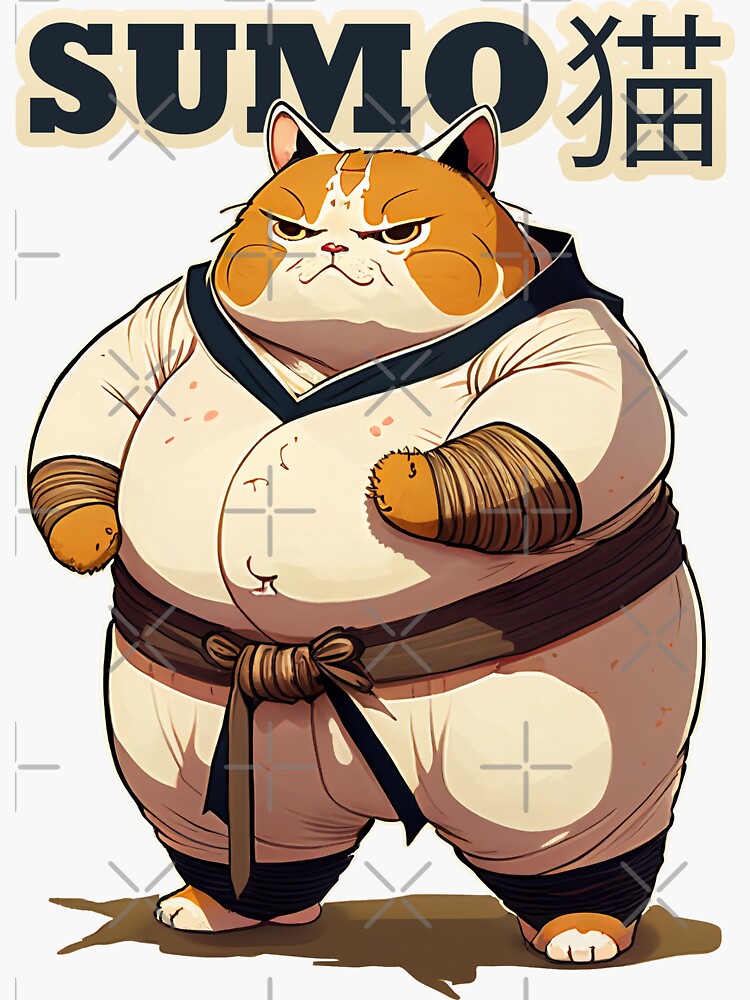The image depicts a comic drawing titled "Sumo," featuring a very large and obese tabby cat with orange and black stripes, and tiny white-marked feet poking out from the bottom. The cat, standing on its hind legs, is dressed in a black belt karate gi made up of shades of brown, tan, and black, indicating it may be a black belt. The cat, with mean eyes, tall ears, and chubby cheeks, strikes a pose as if preparing to fight. The background of the image is light beige, but there are watermarked X's across the screen and the cat casts a brown shadow below. The title "Sumo" and a Japanese word are both written in black font on a yellow background at the top right of the image. The entire scene gives off a mix of a fierce yet somewhat cute aesthetic, reminiscent of an anime or Pokemon style.